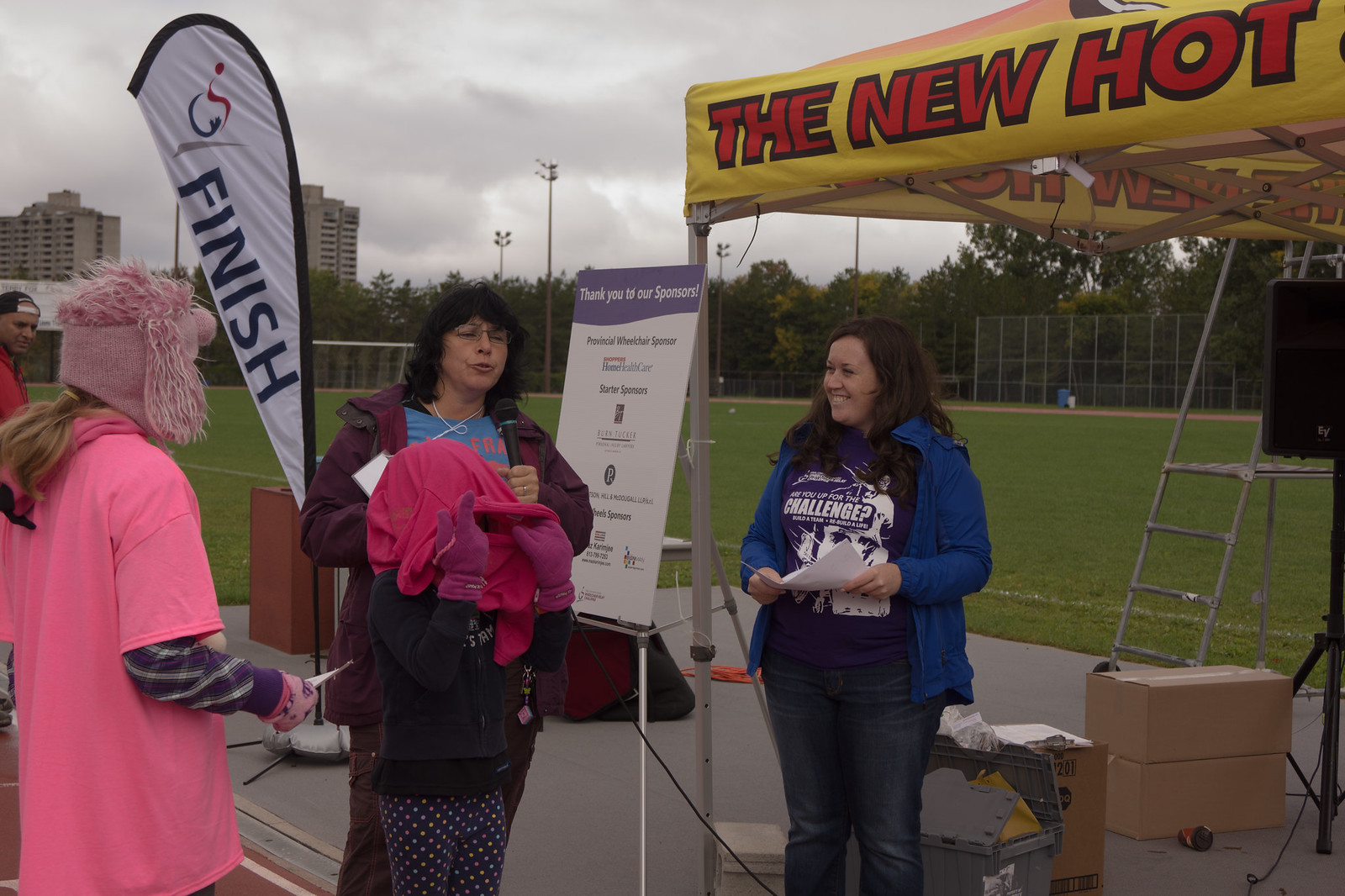In the image, three women are standing in front of a tent with a yellow roof and red text that says "The New Hot" outlined in black. To the right, a woman in a red jacket and a purple shirt that reads "Challenge?" is holding white papers near her stomach. She is dressed in blue jeans and has long brown hair. Next to her is a woman with dark black curly hair, wearing glasses and her eyes closed. She is dressed in a purple jacket over a blue shirt. In front of her is a child wearing black polka dot leggings, a black sweater, and an orange sweatshirt draped over her head, concealing her face. The child is also wearing purple gloves. To the far left, there is a person in a bright pink shirt with a hat featuring dog ears, also pink, and yellow hair showing from the back of the hat. She has purple plaid sleeves and is holding a white object pointing towards the child. 

In the background, a banner on the upper left reads "Finish" in blue letters, and another banner behind the central lady, purple on top and stating "Thank you to our sponsors" with a list of sponsors too small to read, can be seen. The setting extends to a grassy field bordered by a chain-link fence, and farther back, skyscrapers and stadium lights are visible under a cloudy gray and white sky. There's also a man with a baseball cap turned backward, partially visible to the far left.